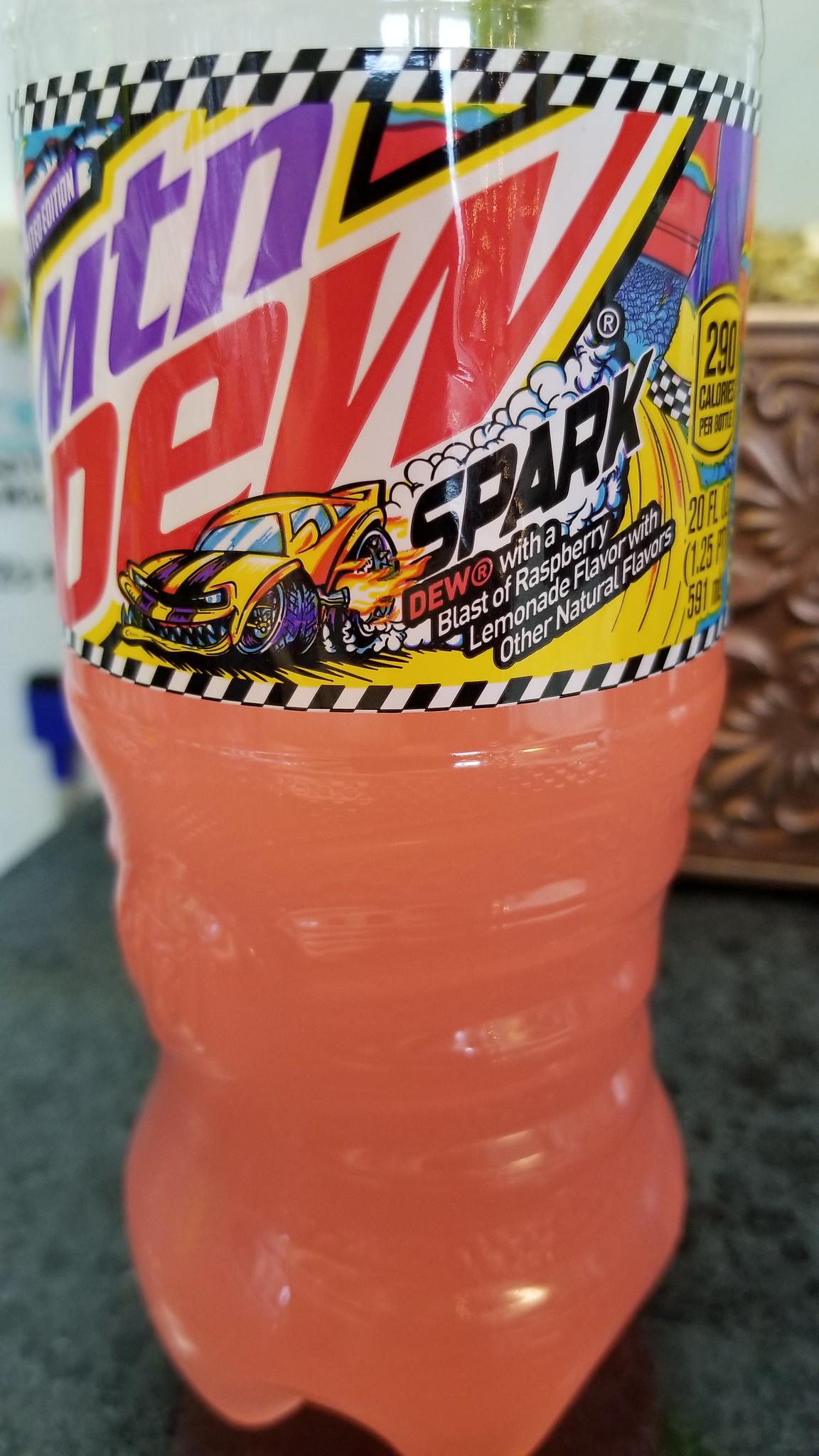A clear plastic bottle is prominently positioned against a gray background. The bottle has various shapes molded into its design and features a bright pink label. The label displays the text "MTN Dew Spark" and describes the drink as "Dew with a blast of raspberry lemonade flavor with other natural flavors." In the background, there is a bird perched above the scene. The image captures a detailed view of the bottle's intricate stencil designs and vibrant colors, providing a focused and visually appealing presentation.